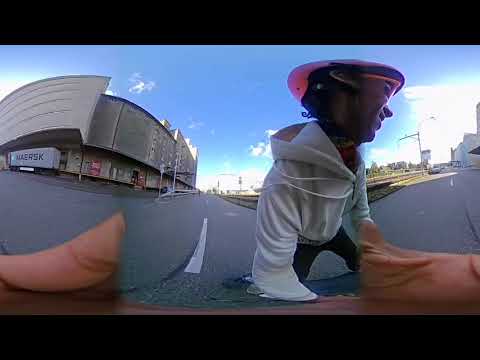This color photograph, bordered in black at the top and bottom, captures a scene with a notable distortion effect likely caused by a specialized lens. The main focus is a person in the foreground, dressed in black pants, a white hoodie, and an orange hat. Their image is slightly warped, particularly at the shoulder and face, which appear exaggerated, while their legs are disproportionately smaller. This individual is looking off to the right and appears to be either kneeling or sitting, although their exact posture is ambiguous due to the distortion.

In the foreground, there is a blurry orange silhouette, possibly of a thumb, adding to the image's surreal quality. The background features a cement driveway or parking lot bordered on the left by a large gray building, which functions as a storage or manufacturing space. Distinguished by some red doors, the building has a visible cargo container labeled "Maersk." To the right of the person, there is a street lined with buildings and cars. The photograph captures a bright, sunny day with a blue sky adorned with puffy, wispy clouds. The overall scene suggests an industrial or commercial setting, with the individual positioned near a warehouse, creating a striking juxtaposition against the expansive sky and urban environment.